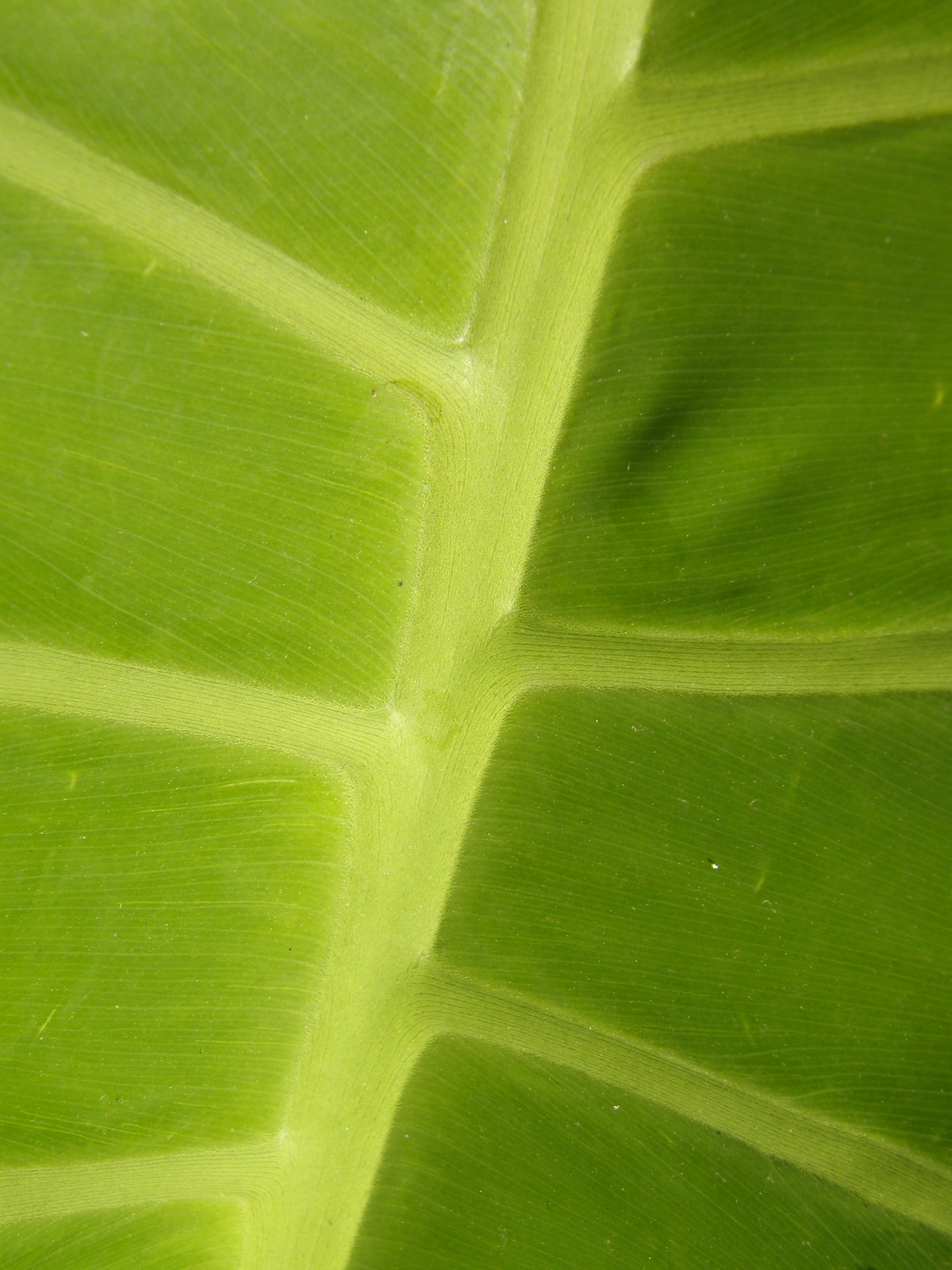This highly zoomed-in photograph captures an intricate view of a leaf from a plant. The leaf is primarily composed of two main colors: a darker green for the main body of the leaf and a lighter green for its veins. On the left side of the image, the leaf appears noticeably lighter, likely due to the way sunlight illuminates this section, resulting in a series of four progressively darker blocks. In the center of the image runs a prominent lighter vein. Extending from this vein are three distinct lines or veins that branch out to both the left and the right, creating a symmetrical pattern. The right side of the photo features four blocks that are darker in comparison to the left. The image contains a consistent green palette, with no other colors, and faint stripes can be observed running parallel along the leaf's structure, possibly suggesting the underside of the leaf is being shown. Overall, the close-up highlights the detailed texture and pattern of the leaf, emphasizing its natural complexity and the distribution of light across its surface.